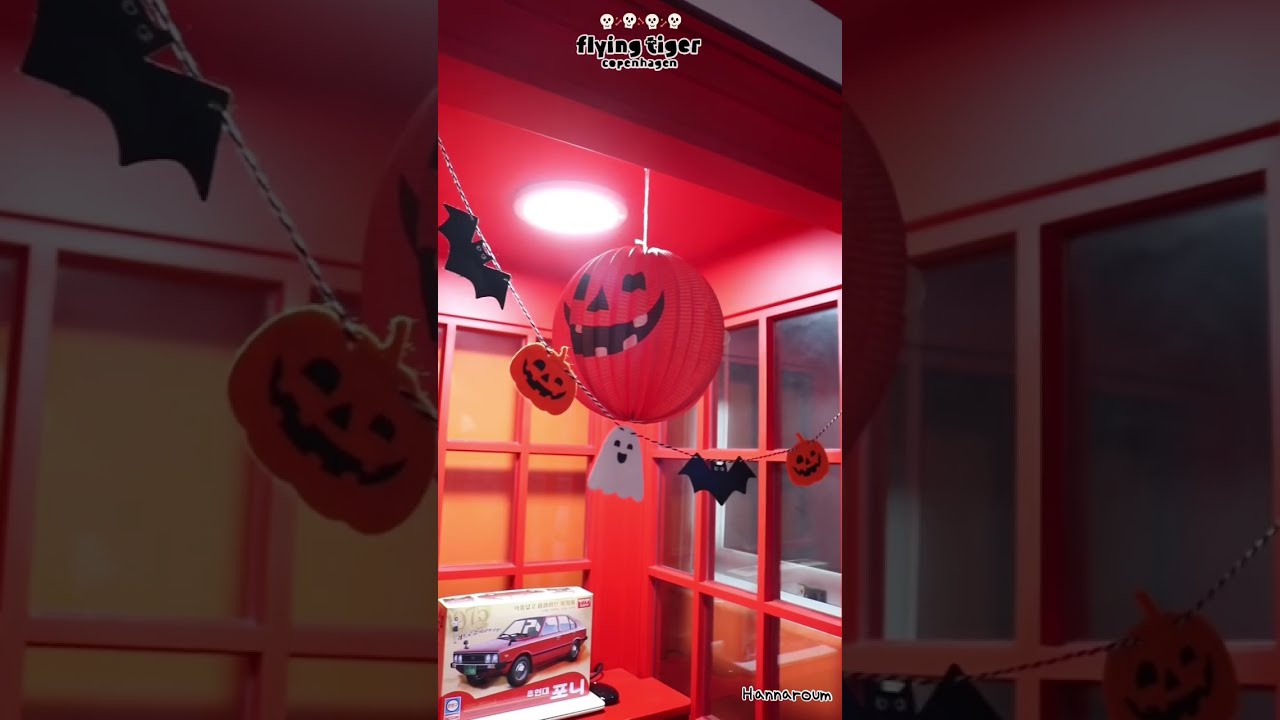This image, likely taken on a phone held upright, captures a vibrant Halloween scene indoors, potentially in a hotel or an establishment affiliated with Flying Tiger Copenhagen, as indicated by text at the top of the image. Dominated by a vivid reddish-orange hue, the room boasts dark wood framing and multiple window panes. The focal point is a large, ball-like pumpkin hanging from the ceiling. Below this centerpiece, a clothesline is strung across the doorway, adorned with small festive decorations, including bats, pumpkins, and a ghost. Despite the Halloween theme, a curious detail at the bottom left corner is a box with an image of a model car on its cover, adding a peculiar touch to the setting. Overall, the room exudes a strong Halloween spirit, emphasized by the brightly lit ceiling and playful decorations.